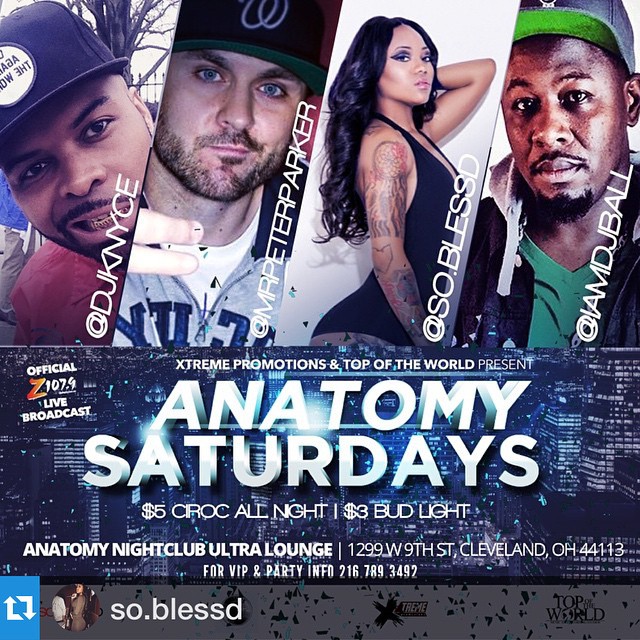The image is a promotional poster for an event called "Anatomy Saturdays" presented by Extreme Promotions and Top of the World. The poster features four individuals, each within angled, rectangular sections. From left to right:

1. A Black man, "@DJKNYCE," wearing a black hat and semi-smiling. He appears to be wearing a red shirt.
2. A Caucasian man, "@MrPeterParker," with blue eyes, a dark beard, and a mustache. He is also wearing a dark hat and shows two fingers in his photograph.
3. An African American woman, "@SOBLESSD," with long black hair, tattoos on her arm, and wearing a tight black dress. She has one hand behind her head and exudes a seductive pose.
4. Another Black man, "@IAMDJBALL," serious-looking, wearing a baseball cap with a green underside and a green V-neck shirt. 

Below these images, a banner displays a cityscape background in blue and black, with the text: "Extreme Promotions and Top of the World Present Anatomy Saturdays." Additional event details include "$5 CIROC All Night," "$3 Bud Light," and the venue information: "Anatomy Nightclub Ultra Lounge, 1299 West 9th Street, Cleveland, Ohio 44113." For VIP and party information, the contact number provided is 216-789-3492. In the lower left-hand corner, there's a small, unclear picture with the text "S.O. Blessed."